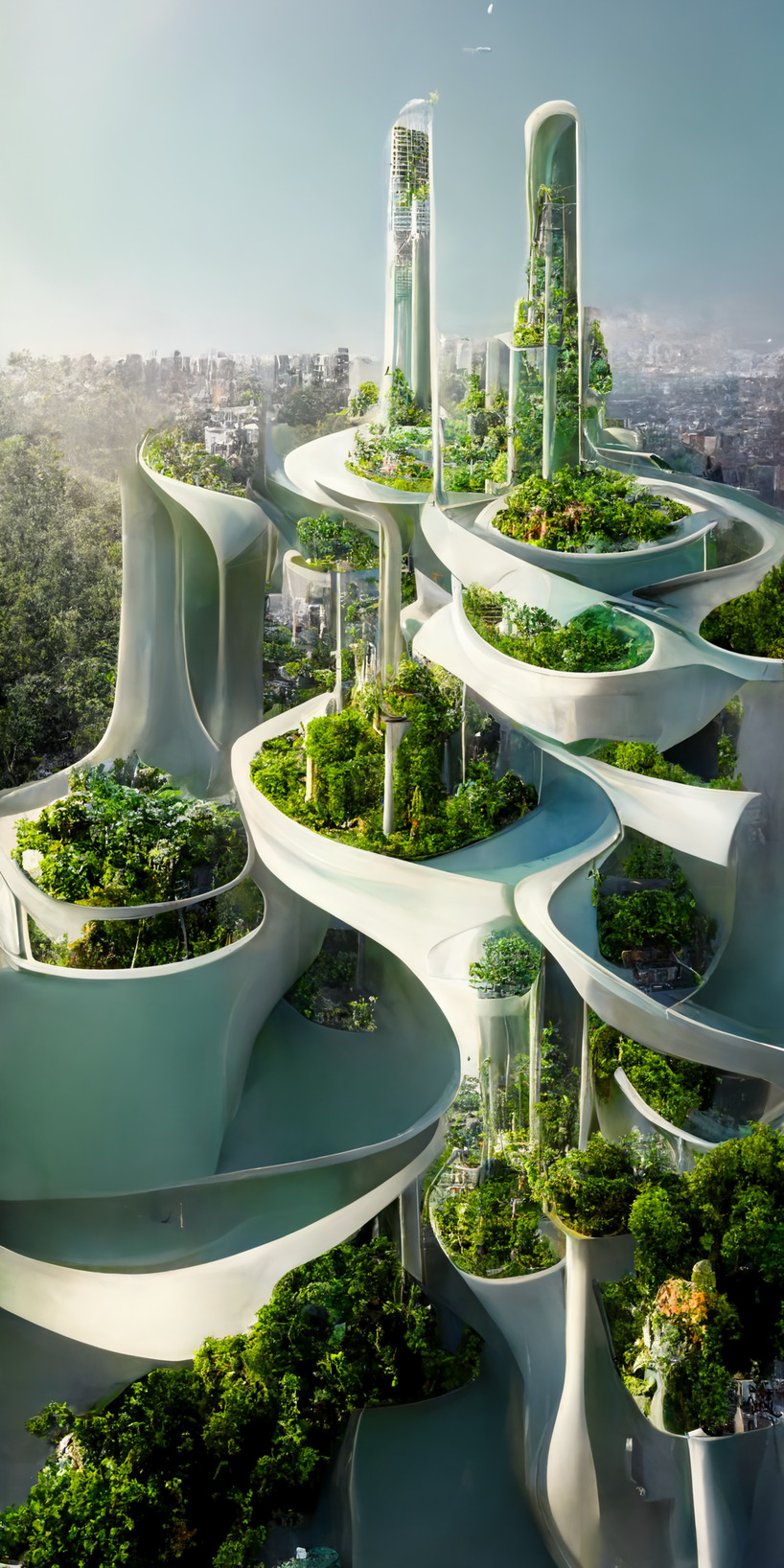The image captures a very tall, futuristic building with an innovative design featuring multiple levels of curved, white balconies serving as greenhouses. Each balcony is adorned with vibrant greenery, including small trees and bushes, giving the appearance of a vertical farm. The ledges have narrow necks that widen outward, creating an undulating profile. The building has two cylindrical tops that also host lush, green plants. In the background, a distant, less distinct city skyline is visible against a clear, blue sky, making the unique architecture of this towering structure stand out prominently. The greenery extends throughout the entire building, including towering capsules filled with plants, contributing to its avant-garde aesthetic. The scene overall presents a blend of urban and natural elements, giving it an otherworldly, almost fictional appearance.